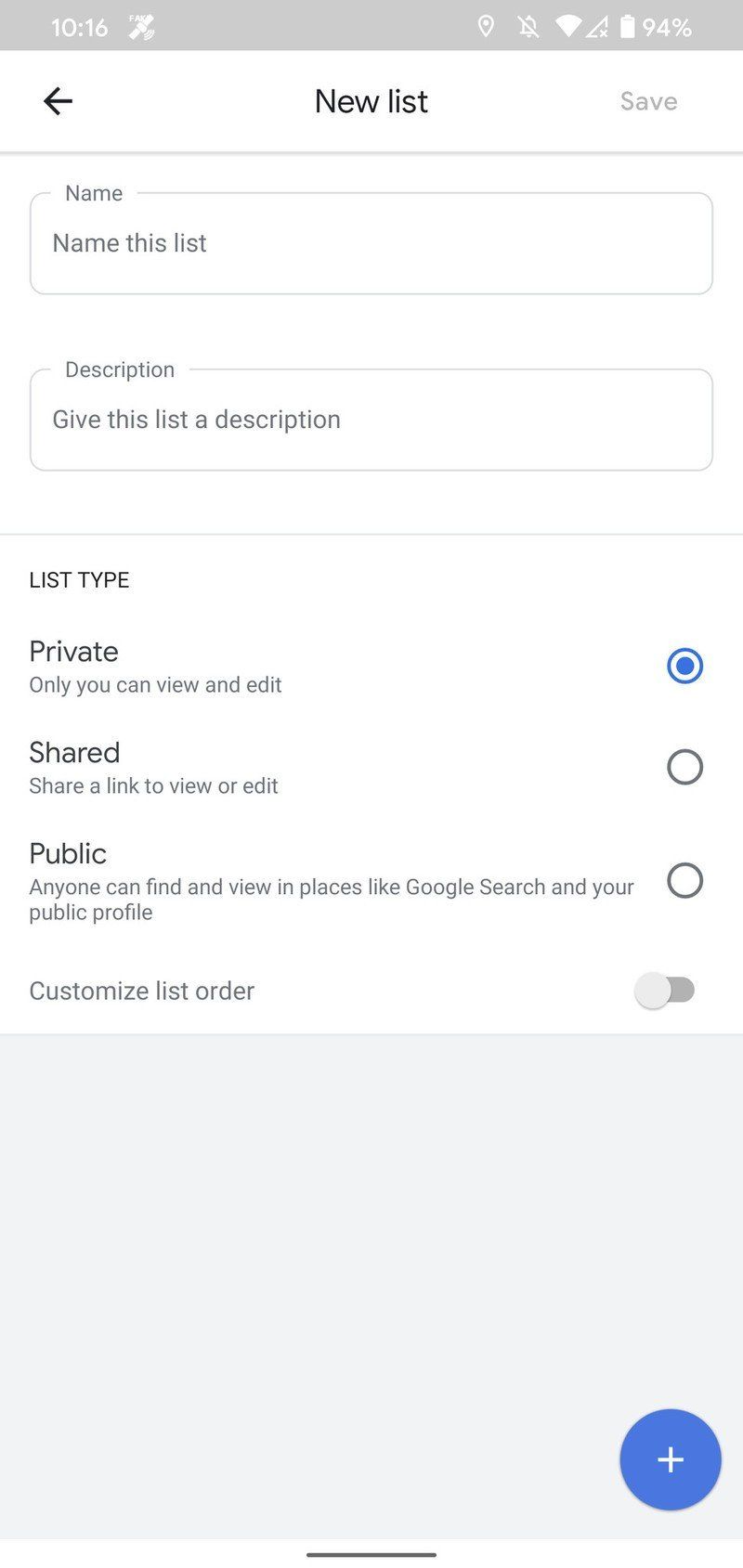The image illustrates an application interface designed for creating new lists. The screen prominently features fields for entering the name and description of the list. Users have the option to categorize the list type as either Private, Shared, or Public. The currently selected option is Private, ensuring lists are kept confidential unless explicitly shared. 

Below these fields, there's an option to customize the list order, though it appears to be disabled, indicated by its dimmed appearance. A plus symbol enclosed within a blue circle is present, which would allow users to add items and rearrange their order once enabled. At the top of the screen, a Save button is available for users to store the list details after they have been entered.